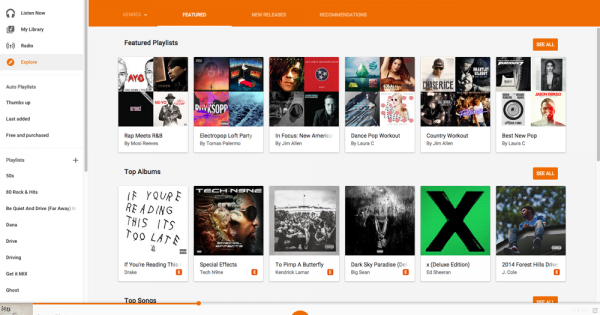This image showcases a comprehensive music streaming interface. The top section features primary navigation icons, including "Listen Now," "My Library," and "Radio." Below these, there are options for exploring music, auto-generated playlists, and a "Thumbs Up" section for favorited songs. Additionally, you can see sections for "Last Added," "Free & Purchased," and other playlist categories like "Drive Driving," "Get a Mix," and "Ghosts."

Towards the bottom of the interface, the screen is populated with various thumbnails and album advertisements. Major categories highlighted include "Top Albums," "Featured Playlists," "New Releases," and "Recommended" selections, visually represented by colorful album covers and promotional images.